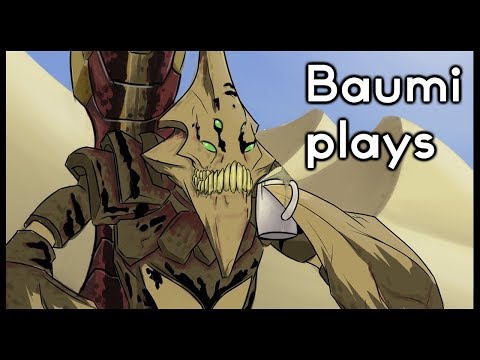This cartoon image, set against a sunny, cloudless blue sky, features a prominent scorpion character front and center. The background showcases a desert landscape with two large, pyramidal-shaped sand dunes made of light tan sand. The scorpion, a multicolored tan alien creature with green slanted eyes — three fully visible and one partially peeking — and a diamond-shaped face lined with large yellow teeth, faces the camera. Its menacing appearance is softened by the white coffee cup it holds in its left claw, which is raised towards its face. The scorpion's long, scaly reddish-tan tail arches over its back, adding to its exotic look. In the upper right-hand corner of the image, the text "Baumi Plays," spelled B-A-U-M-I, appears in white with a black border, providing a playful caption to this whimsical yet intriguing scene. The entire image is bordered by a horizontal black rectangle, thicker at the top and bottom and thinner on the sides.